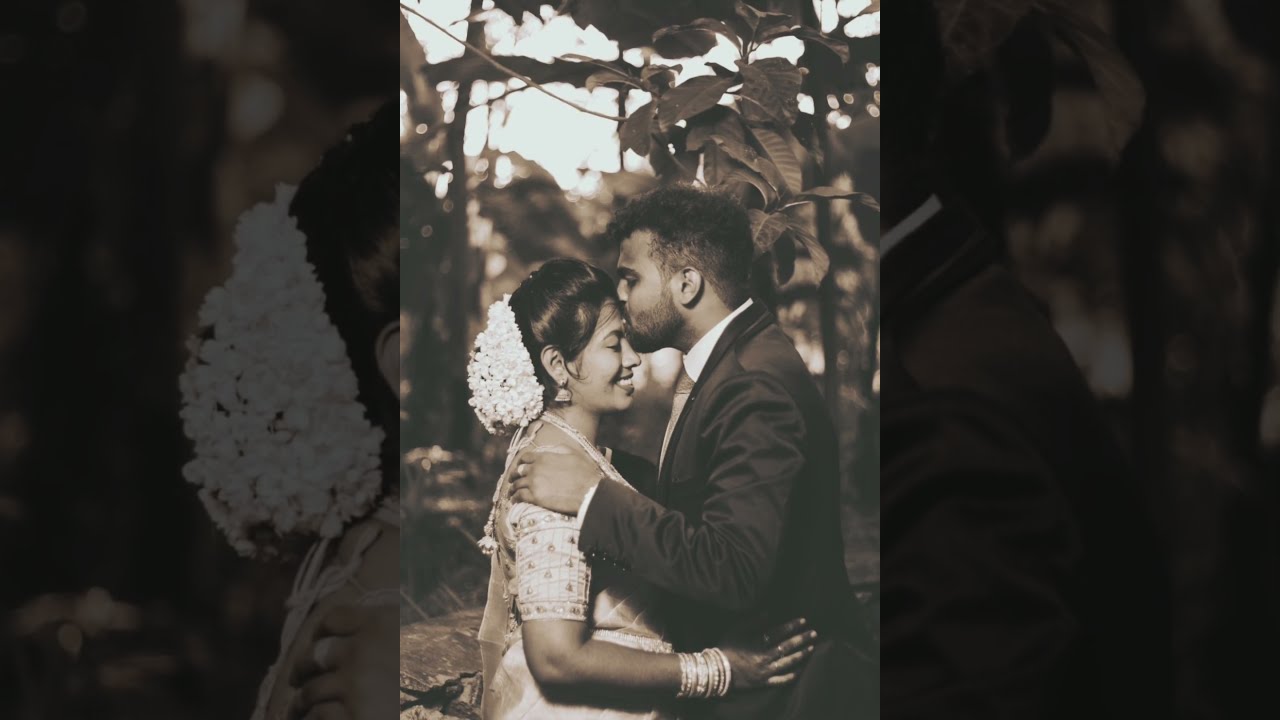This grayscale photograph captures a tender, intimate moment between a bride and groom, possibly of South Asian descent, on their wedding day. The groom, who has short dark curly hair and a close-shaven beard, is lovingly kissing the bride on her forehead, his hands resting gently on her shoulders. The bride, adorned with white flowers in her dark, pulled-back hair, is smiling warmly. She is dressed in an intricately designed traditional wedding dress, heavy with beadwork, and accessorized with multiple bracelets and earrings. Her hands are placed tenderly on the groom's waist. They are standing outdoors in front of lush, large-leafed plants. The bride appears on the left while the groom is on the right in this portrait-oriented photograph. The image has been artistically presented, with semi-transparent black layers on either side, magnifying the bride's floral hair arrangement on the left and the groom's suit detail on the right, creating a harmonious, landscape-oriented composition.